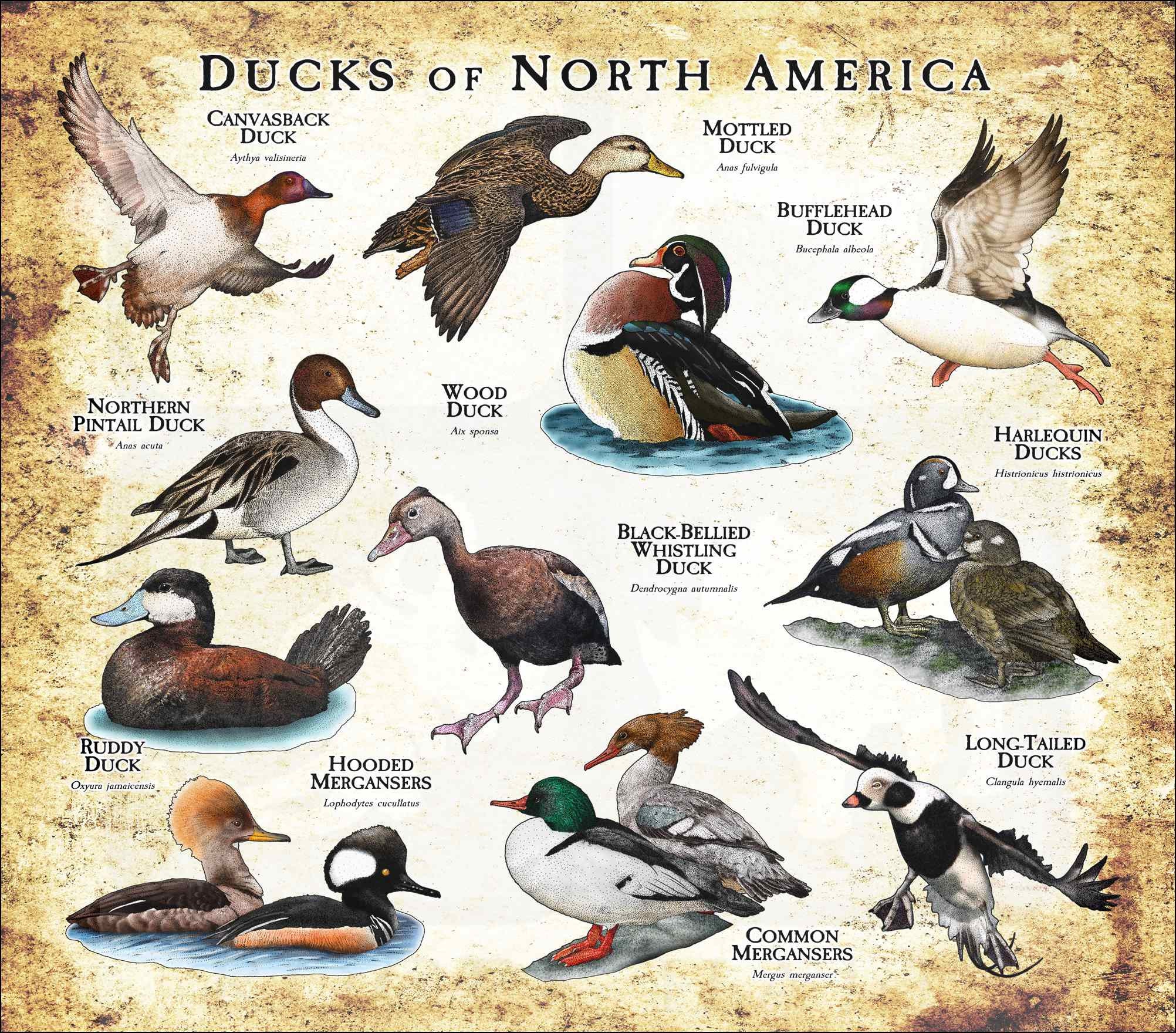This poster, titled "Ducks of North America," is a detailed illustration featuring approximately 11 different species of North American ducks. The background is predominantly white with a beige, sand-colored border that has an uneven, textured pattern reminiscent of old parchment. The title is prominently displayed at the top in a standard font.

The ducks are arranged in a grid format, starting from the top left and labeled both in English and their respective scientific names, although the latter are too small to read clearly. The species listed on the poster include:

1. Canvasback Duck
2. Mottled Duck
3. Bufflehead Duck
4. Wood Duck
5. Northern Pintail Duck
6. Black-bellied Whistling Duck
7. Harlequin Duck
8. Ruddy Duck
9. Hooded Merganser
10. Common Merganser
11. Long-tailed Duck

Each duck is depicted in various poses, with some in flight and others floating or grooming in the water. The illustrations showcase a diversity of colors such as gray, blue, black, maroon, green, and pink, which highlight the unique plumage of each species. This poster serves as a visual guide to the ducks of North America, reminiscent of the detailed naturalist drawings found in classic birdwatching books.